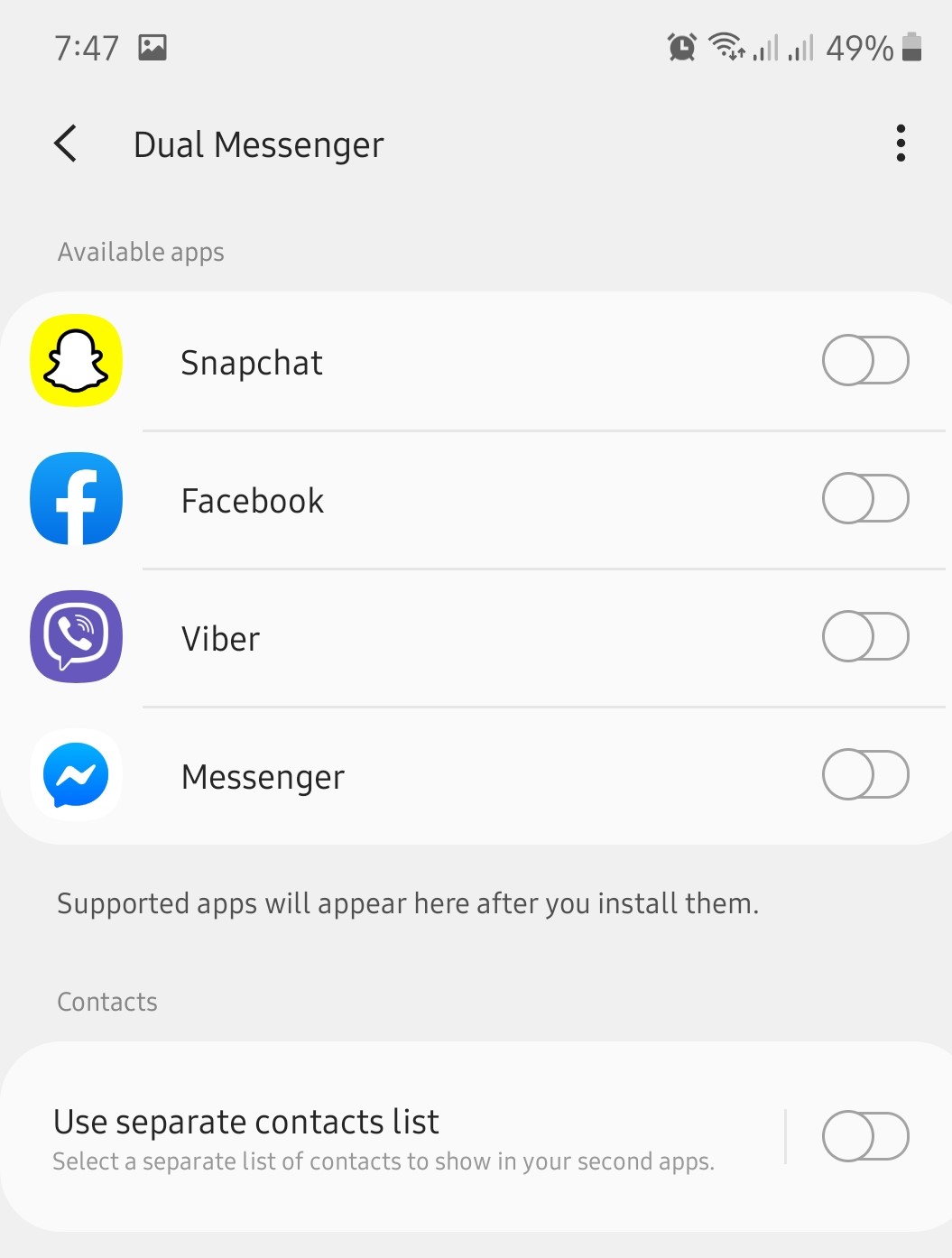In this image, you see a detailed screenshot of a mobile device interface. At the top left, the time displays as 7:47. The gallery notification icon is also visible. Moving to the top right corner, there are several status indicators: an active alarm icon, a Wi-Fi signal strength icon showing a full four out of four bars, and two network signal indicators, both showing two out of four bars. The battery level is at 49%. Beneath these indicators, the page content shows "Dual Messenger" and lists available apps such as Snapchat, Facebook, Viber, and Messenger. The message indicates that supported apps will appear here after installation. There is also an option to use a separate contact list, which is currently not selected.